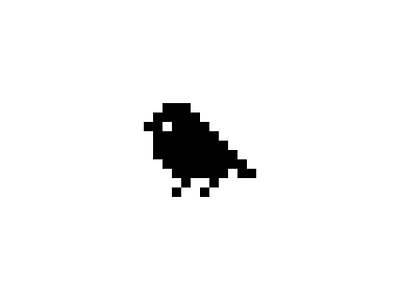This image is a small, simplistic pixel art representation of a bird rendered entirely in black on a pure white background. The bird is composed of blocky, pixelated shapes, reminiscent of early video game graphics. The head is crafted from three black pixels with a single white pixel representing its eye. The beak is only one pixel, and its legs are two pixels each. The bird features a straight, rigid tail roughly five pixels long, extending at a 45-degree angle. Its body tapers with a staircase-like pattern, both on the back and front, creating a jagged outline. The entire image is devoid of any text or color besides the black and white, offering high contrast and a primitive, retro aesthetic. The bird faces left, away from the viewer, contributing to its minimalist charm.